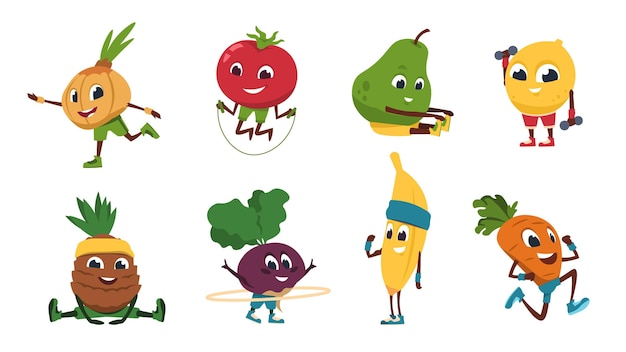This is a colorful and lively cartoon image featuring ten anthropomorphic fruits and vegetables, all engaged in various exercises against a white background. Each character, designed with expressive faces and cute eyes, is busy performing a different physical activity:

1. A carrot with blue shorts, green hair, and blue shoes is shown sprinting energetically.
2. A red tomato with a green stem and green shorts is joyfully jumping rope.
3. A green pear dressed in yellow pants and shoes sits on the ground, stretching to touch its toes with a happy smile.
4. A yellow lemon, wearing pink shorts and red shoes, is depicted lifting two weights, showcasing its strength.
5. An enthusiastic onion with an orange face and green slacks is depicted running.
6. A cheerful banana adorned with a green headband, wristbands, and blue shoes is flexing its bicep with a big grin.
7. A pineapple with green pants and a stem, sitting with legs spread, appears to be stretching.
8. A green-haired character with green shorts, possibly a melon or tangerine, stands with outstretched arms.
9. A purple radish donned in green shorts and shoes is actively hula hooping.
10. A brown potato or coconut, wearing green shoes, seems to be in a stretching pose.

Each character's vibrant colors and detailed attire, such as headbands, wristbands, and variously colored shorts and shoes, add to the playful and dynamic scene, emphasizing a theme of fun and fitness.